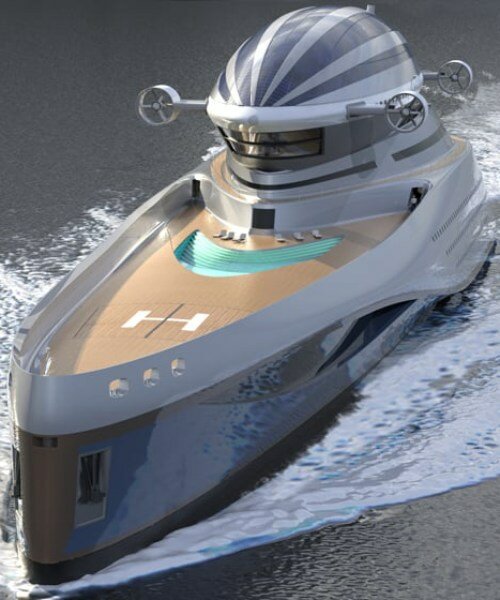The image is a highly detailed and realistic-looking computer-animated illustration of a unique superyacht in speed, set in a portrait style and in full color. The yacht, which is primarily silvery-gray with a wooden light brown deck, showcases several unusual features. At the front of the vessel, there's a helipad marked with a white 'H'. Centered on the deck is a pool with a very light blue water hue, surrounded by pool chairs. 

One of the standout characteristics of this superyacht is the large dome-like structure located towards the back. This dome appears to be equipped with four propeller-like fans, suggesting it might be designed for submersible capabilities, although its exact function is not entirely clear. The water around the yacht is a gray color, mirroring the vessel’s sleek appearance. Despite appearing small, which might suggest it could be a miniature or radio-controlled model, the meticulous detailing points to a cutting-edge design in yacht engineering.